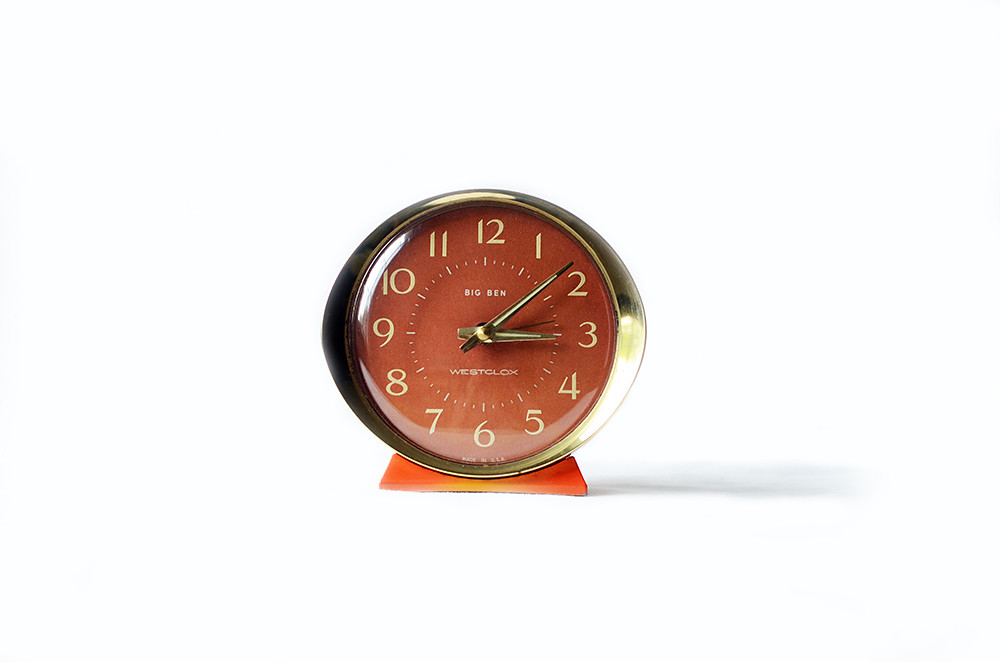This image features a classic bedside clock with a round, metal bronze frame. The clock's face is white, adorned with distinctive yellow-gold numbers. Below the 12 o'clock mark, the brand name "Big Ben" is prominently displayed in white font. Circular lines encircle each number, adding an element of intricate detailing. The clock hands, pointing at the time, are attached to a central point labeled "Westclox." The clock rests on a square base, which is a subtle blend of light orange and yellow hues, complementing the bronze frame and adding a touch of warmth to its overall appearance.